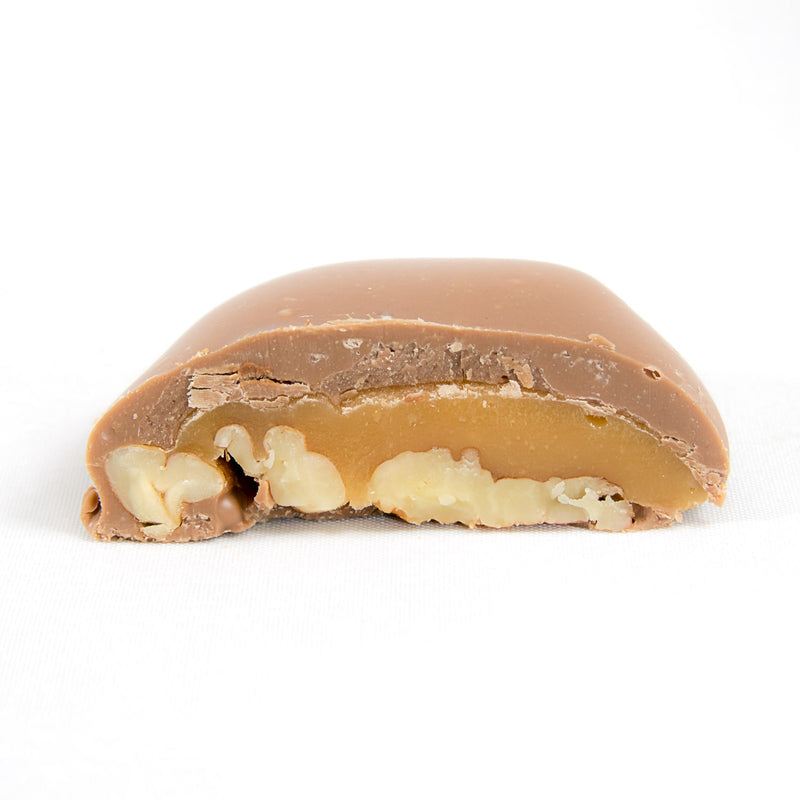This professionally taken, well-lit photograph features a close-up of a uniquely colored candy bar against a white background. The candy bar has been sliced to reveal its detailed, multi-layered interior. The topmost layer appears to be a pale milk chocolate, distinctively tan rather than typical dark or white chocolate. Below this chocolate coating lies a sticky, firm caramel layer with a rich orange-yellow hue. The bottom layer seems to consist of what looks like ground nuts or seeds, possibly walnuts or peanuts, characterized by an off-white to light brown shade. The image lacks any branding or text, allowing the focus to remain on the enticing textures and colors of the three distinct layers: the smooth tan chocolate, the glossy caramel, and the nutty or seedy base.